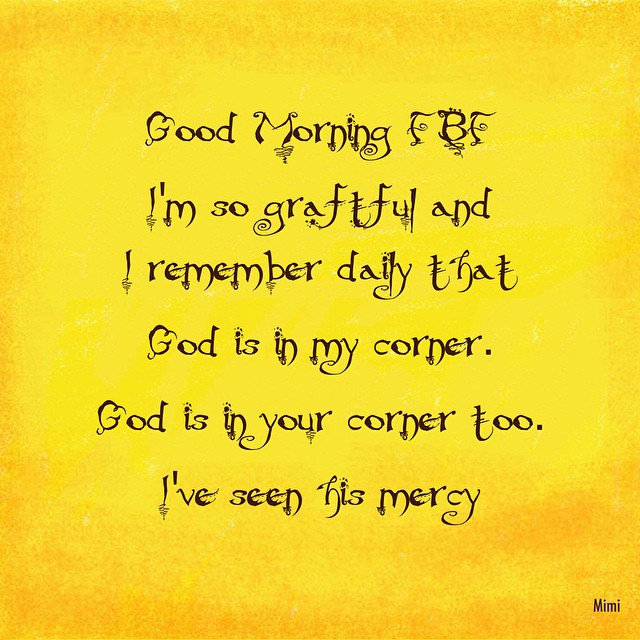The image features a gold and yellow background with varying shades; it darkens ever so slightly at the very top and bottom, while the middle is the brightest. The main text, written in a highly stylized, almost gothic or Tim Burton-esque black font that resembles handwriting, reads: "Good Morning, FBF. I'm so grateful, and I remember daily that God is in my corner. God is in your corner too. I've seen His mercy." At the bottom right corner, "Mimi" is written in small, regular black block letters, suggesting either the creator or the attribution of the quote. The detailed interplay of gold and yellow, along with the intricate font, adds a striking visual appeal to the image.